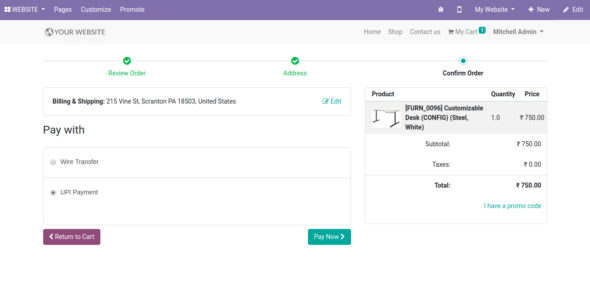Screenshot of Shipping Page – The screenshot features a website interface predominantly highlighted with a purple navigation bar spanning the top from left to right. This bar contains various options, such as "Website Pages," "Customize," "Promote," "My Website," and "Edit." An additional reminder in gray text at the upper section prompts users to "See Your Website."

Despite the slightly grainy image quality, the top right corner clearly displays further navigation options including "Home," "Shop," "Contact Us," and "My Cart (1)." The logged-in user is identified as "Mitchell Admin."

In the main content area, a step-by-step view of the order process lists stages: "View Order," "Address," "Confirm Order," and "Billing and Shipping." The specific address shown is 215 Vine Street, Scranton, Pennsylvania, 18503, United States. The payment method is stated as "Wire Transfer," with the shipping method listed as "UPS Payment."

On the left-hand side of the screenshot, there’s a prominent pink button labeled "Return to Cart" in white text. Mirrored on the right is a green button with the text "Pay Now," also in white.

The right-hand side of the image showcases the product being ordered: a "Ferno 096 Customizable Desk" in a steel white finish. Details include a quantity of 1 piece, priced at 750 rupees. The subtotal is 750 rupees with no additional taxes applied, summarizing the total cost to 750 rupees.